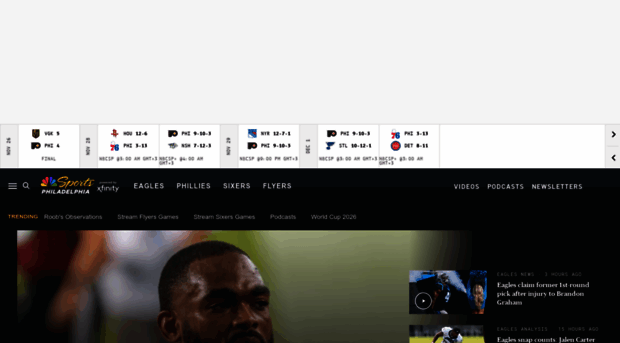This image is a cropped screenshot of sports scores displayed on a website. At the top of the page, a broad, empty light gray rectangle spans the full width of the screen. Below this section is the main area containing the scores, which is set against a white background. On the right side of the screen, there's a light gray rectangle divided by a thin light gray vertical line, which splits the rectangle into two; the upper section features a black arrow pointing to the right, while the bottom section has a black arrow pointing to the left. To the left of this divided rectangle lies a broad expanse of negative space.

Within the main area of the page, there are alternating boxes of scores and dates. The scores are displayed in white boxes outlined with light gray lines and feature team logos in the top left and bottom left corners. Dark gray text indicating the scores is positioned to the right of the logos. Additionally, there is light gray text at the bottom of each score box. The dates are presented in a vertical orientation within light gray boxes, with medium gray text.

Beneath the scores section is the website’s header. The header includes a bluish dark gray rectangle at the top, followed by a black section underneath. The header text is placed such that it intersects both the header background and the page background. On the left side of the header, there is a white hamburger menu icon, followed by a magnifying glass icon slightly to the right. Further details are present beyond these icons, continuing to the right.